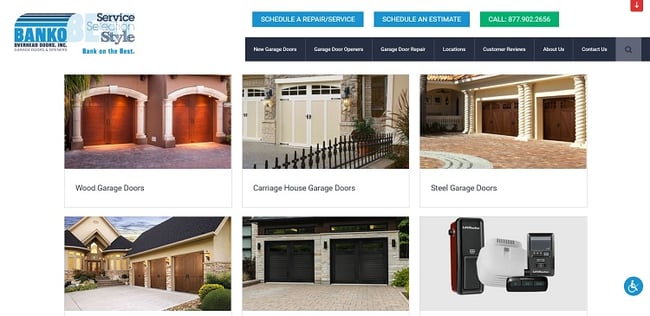The image features a white background with a blue logo in the upper left corner that reads "Banco Service Selection Style." Across the top, there are a series of buttons: a blue button with white text that says "Schedule a Repair Service," another blue button with white text that reads "Schedule an Estimate," and a green button that says "Call" accompanied by a phone number. Beneath these buttons, there's a black banner with white text listing several options: "New Garage Doors," "Garage Door Openers," "Garage Door Repair," "Location," "Customer Reviews," "About Us," and "Contact Us." 

Below this banner, the image displays six color photographs. The top row features three labeled images of different types of garage doors: "Wood Garage Doors," "Carriage House Garage Doors," and "Steel Garage Doors." The bottom row contains three unlabeled images, two showcasing the fronts of garages and one displaying equipment related to garage doors.